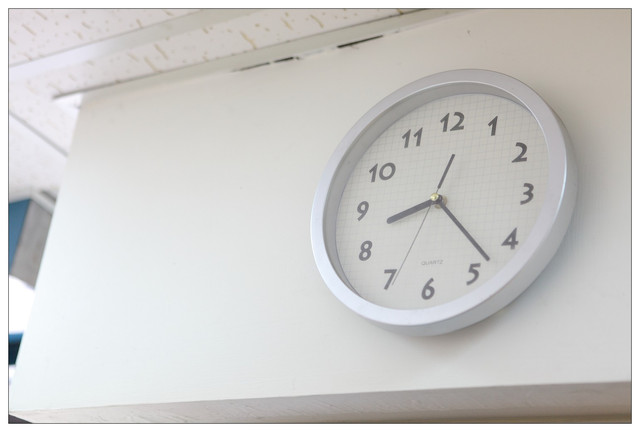A white wall clock is mounted on a protruding structure near the ceiling of a room. The clock features a sleek, white rectangular design that complements its plastic or metal rim. The ceiling nearby consists of gray-streaked, white ceiling tiles. The clock face is unique, resembling graph paper with faint blue-lined squares overlaying a white background. This minimalist design lacks the typical hour markers or finer lines usually seen between numbers, giving it a clean and modern look. The white dial, adorned with plain numerals, indicates the time as 8:23.